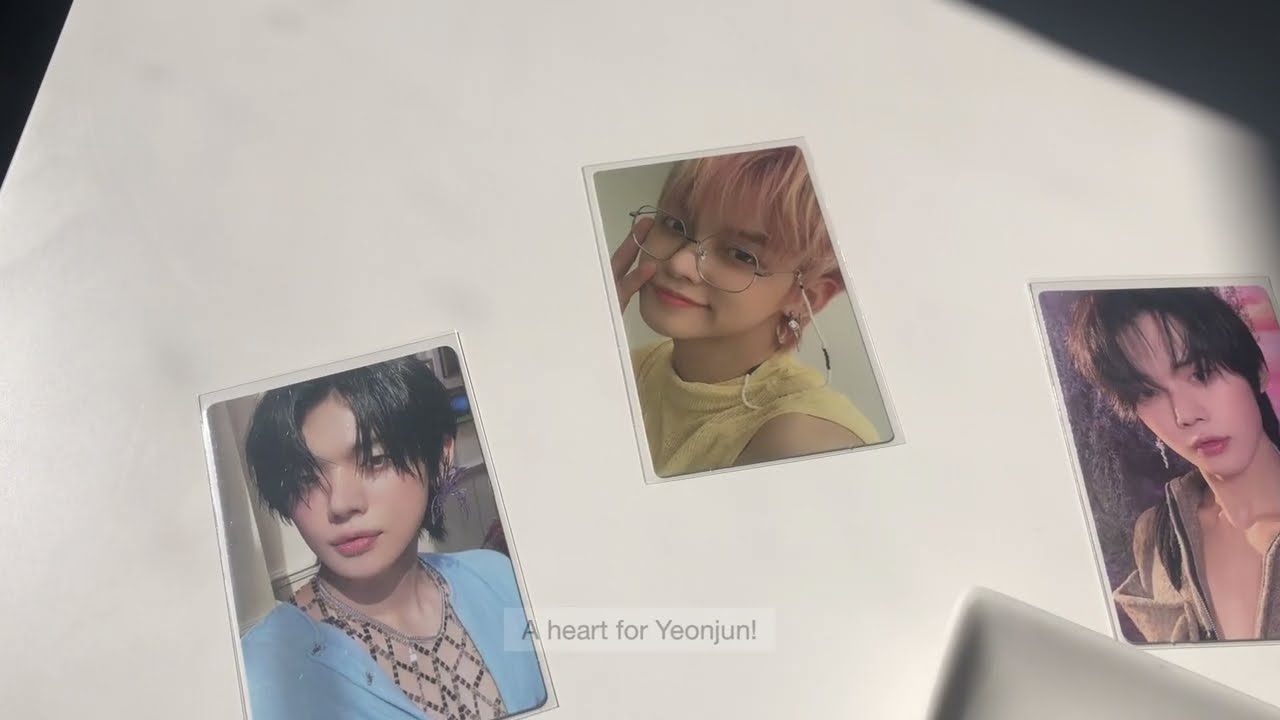The image consists of three Polaroid-style photographs arranged on a white surface, possibly a table or a wall, with the surface remaining ambiguous. The photos are placed in a row with slight counterclockwise tilts and depict a young woman of Asian descent, styled differently in each image. 

- The left photo shows her with short black hair, partially covering her eyes, and wearing a blue cardigan over a top that resembles chain mail. The caption "A heart for Yujin" is written next to her in black font.
- The middle photo features the same young woman, this time with light brown hair and circular eyeglasses. She is dressed in a sleeveless yellow tank top and has one hand touching her face.
- The right photo again shows the woman with short black hair, styled to be shoulder-length at the back and ear-length at the front, with visible earrings. She is wearing a gray jacket that has a slightly revealing neckline.

Overall, the background remains uniformly white, providing a clean and simple backdrop for the detailed and varied portraits of the young woman. The images include subtle personal touches, such as the handwritten messages, which suggest an intimate and affectionate context.